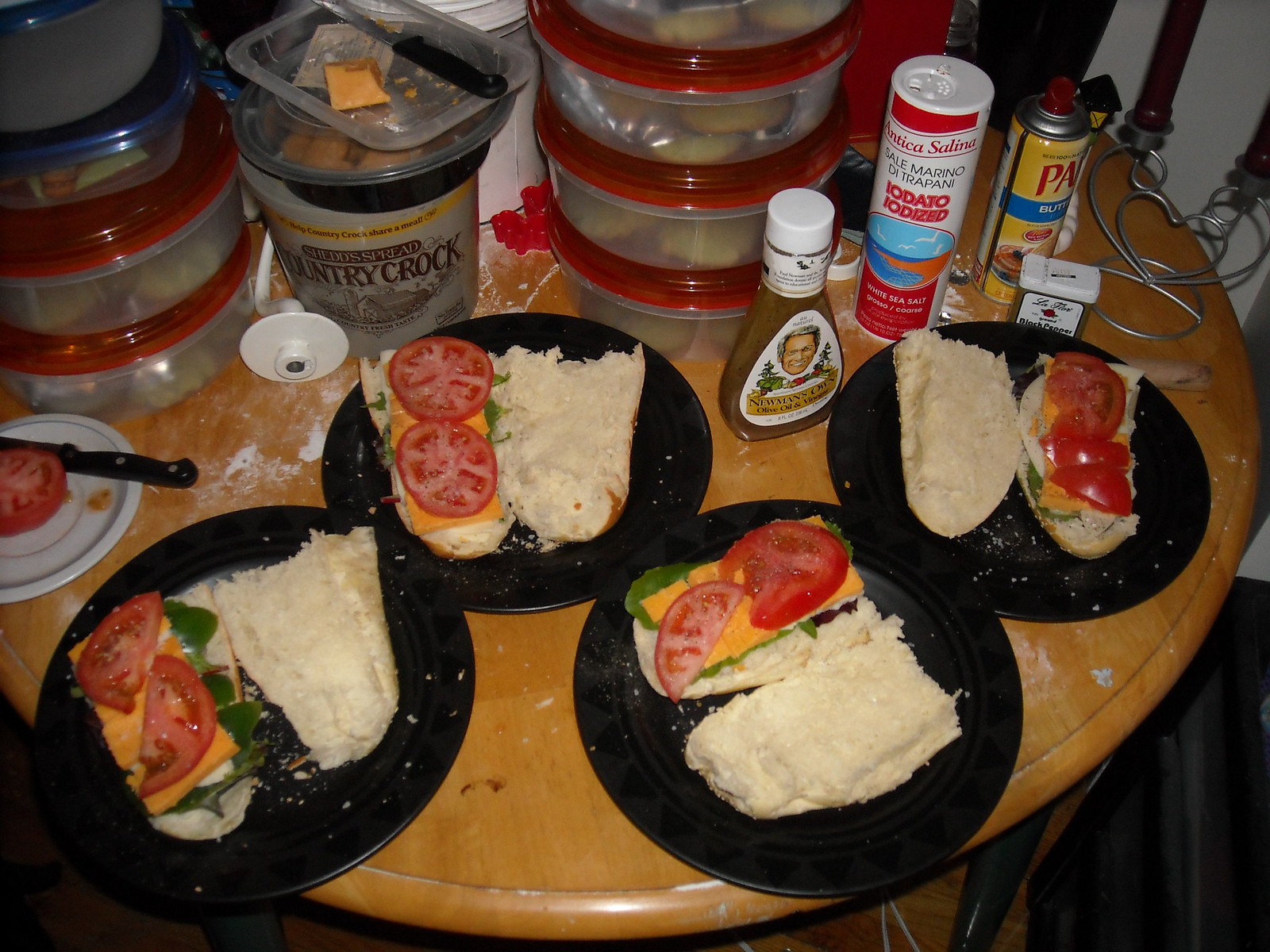The amateur photograph depicts a cluttered round wooden table with four black plates precariously crammed together, each holding messy open-faced sandwiches. Each sandwich is topped with fresh ingredients, prominently featuring tomatoes, cheese, and lettuce, seasoned with salt and pepper. The table is a chaotic scene, surrounded by an array of additional ingredients and kitchen items. There is a bottle of Newman's Own olive oil and vinaigrette salad dressing, a container of Country Crock butter, a white plate with sliced tomatoes, and a knife resting across it. Pam cooking spray and another container labeled iodized salt also occupy the limited space. In the background, stacks of clear Tupperware containers with white lids are visible, some holding what appear to be cookies. To the side, a quaint candelabra with two wicks adds a unique touch to the otherwise hectic setting. The table is set against a wooden floor, contributing to the rustic atmosphere of the image.